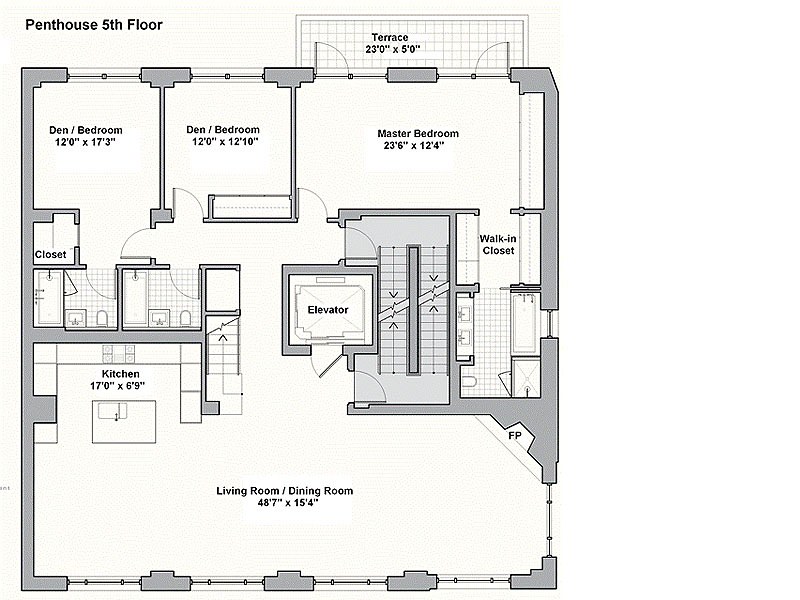This computer-generated floor plan represents a penthouse located on the fifth floor. The layout is depicted on a white background and features a square structure with detailed room allocations and measurements.

At the bottom of the plan, there is a combined living room and dining room area, which includes a kitchen nestled into a nook in the top left corner of this space. The kitchen has a U-shaped design with an island at the center, housing the sink. The stove is mounted on the wall that serves as a boundary to the adjacent rooms. Adjacent to the living area, in the upper right corner, is a fireplace (designated as FP) placed catty-cornered. This area is well-lit with four windows along the bottom side and one window to the right of the fireplace.

To the right of the kitchen, a stairwell provides access to different floors. Next to the stairwell, there is an elevator, accompanied by a hallway that separates them. Another stairwell is located to the right of the elevator.

Behind the kitchen, there are two bathrooms. One bathroom has dual access, with doors leading into the hallway and a den/bedroom situated in the upper left corner. The second bathroom, equipped with a bathtub, is connected to a closet within the den/bedroom area.

The penthouse includes several sleeping and multipurpose rooms: two potential den/bedrooms and a master bedroom located in the upper right corner. The master bedroom features dimensions of 23 feet 6 inches by 12 feet 4 inches and offers access to a private terrace through two French doors. Attached to the master bedroom is a walk-in closet, leading into an en-suite bathroom outfitted with a shower, a bathtub, and a double sink countertop.